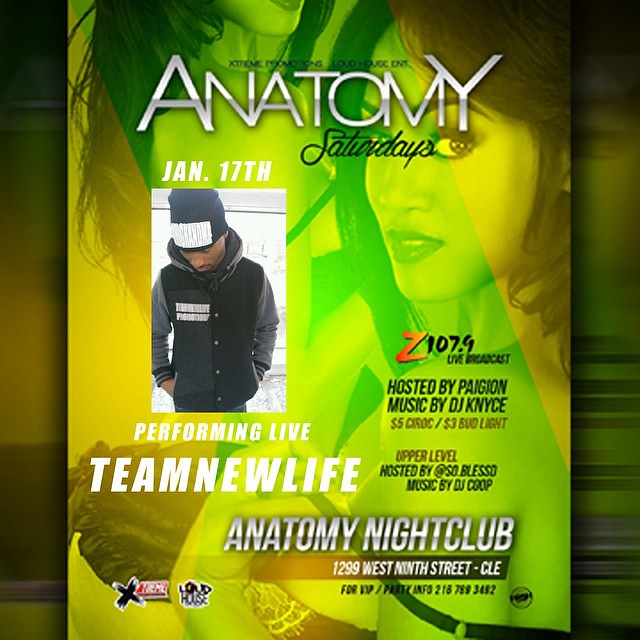The image is a vivid, colorful flyer for a nightclub event. The background features green, blue, and gold shades with a prominent image of a woman, possibly two different angles or two women, both with dark hair. One woman is looking into the camera, turning her head, while the other is pulling down her bra. At the top of the flyer, the text "Anatomy Saturdays" is written in silver-white lettering, with "January 17th" just below. There is also a picture of a man, head down, wearing a black jacket and hat. Below his image, the text reads "Performing Live, Team New Life."

On the right side, it states "Z107.9 Live Broadcast" hosted by Pygon, with music by DJ KNYCE. The flyer also advertises $5 Ciroc and $3 Bud Light drinks. The upper level of the event will be hosted by So Blessed, with music by DJ Coop. At the bottom of the flyer, in silver letters, it reads "Anatomy Nightclub, 1299 West 9th Street, CLE," and beneath that, in black text, "For VIP/Party Info: 216-789-3452." Additionally, the logos for the sponsors Extreme and Loud House appear in the bottom corners.